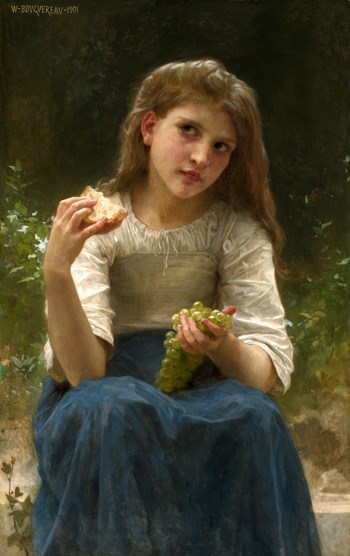This is an exceptionally realistic and colorful painting of a young, contemplative girl sitting on the edge of a white stone or wall. She appears to be around 12 years old, with light to medium brown hair that has a slight wave and is pushed back behind her right ear. She is dressed in a long blue skirt and a white frilly shirt with sleeves that extend to her elbows. The girl holds a bunch of green grapes in her left hand and a partially eaten piece of white crusty bread in her right hand. She tilts her head slightly to the left, gazing up and to the right with a serious, thoughtful expression. The background is lush with green leaves, some green vines to her side, and a gradient that shades towards dark black at the top. There are also small white flowers interspersed among the greenery. The artist's signature is unobtrusively placed in the upper left-hand corner of the painting.